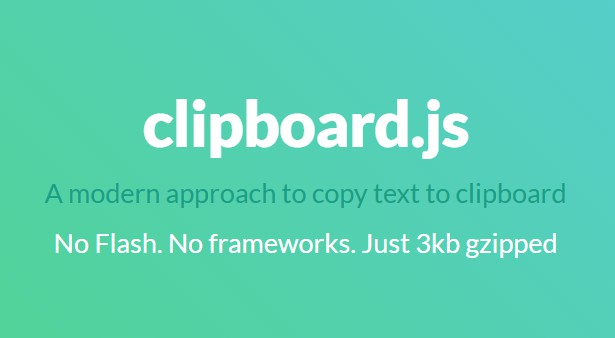The image features a bluish-green rectangle with white and gray text arranged in a clean, modern format. At the top of the rectangle is "clipboard.js" in a large, bold, all-lowercase white font. Below this, in smaller gray text, it reads, "A modern approach to copy text to clipboard," with the sentence beginning with a capital "A." Further down, in three separate lines, the text states: "No Flash." followed by "No frameworks." and then "Just 3 KB gzipped." Each of these phrases starts with a capital letter and ends with a period. The phrases "No Flash.", "No frameworks.", and "Just 3 KB gzipped." are also in white text, matching the style of "clipboard.js." The overall design emphasizes the simplicity and efficiency of the clipboard.js feature.